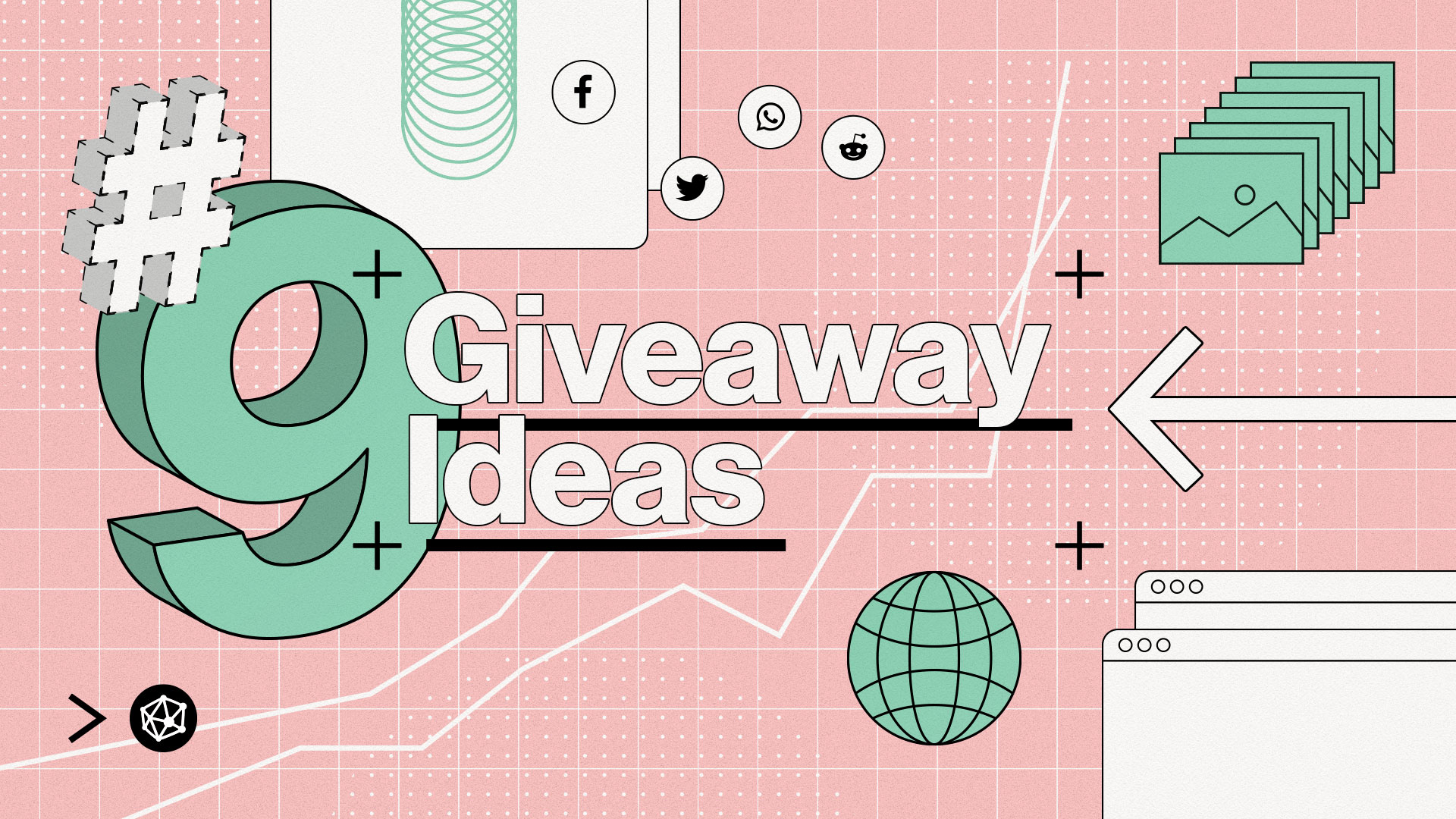The image features a vibrant pink background adorned with white grid lines and dots, giving it a structured yet dynamic appearance. Prominently displayed in the top left corner is a three-dimensional white hashtag (#) symbol, followed by a substantial green number 9 with a black outline, also rendered in 3D. Centrally positioned is the phrase "Giveaway Ideas" in bold white text, underlined in black, accompanied by a black arrow pointing to the left.

Adding to the graphical richness, the top section hosts a square featuring green circles, while nearby, social media icons for platforms such as Facebook, Twitter, Instagram, and WhatsApp are displayed within green circles. To the right, there is a stack of green image symbols, reminiscent of the Microsoft photo file icon. A green and black globe, echoing the classic internet symbol, is situated at the bottom. The image also includes a distinctive white section in the bottom right corner. 

Collectively, these elements form a cohesive, eye-catching digital graphic, likely designed to illustrate "Nine Giveaway Ideas" for an article or online content, artfully combining social media and digital themes.